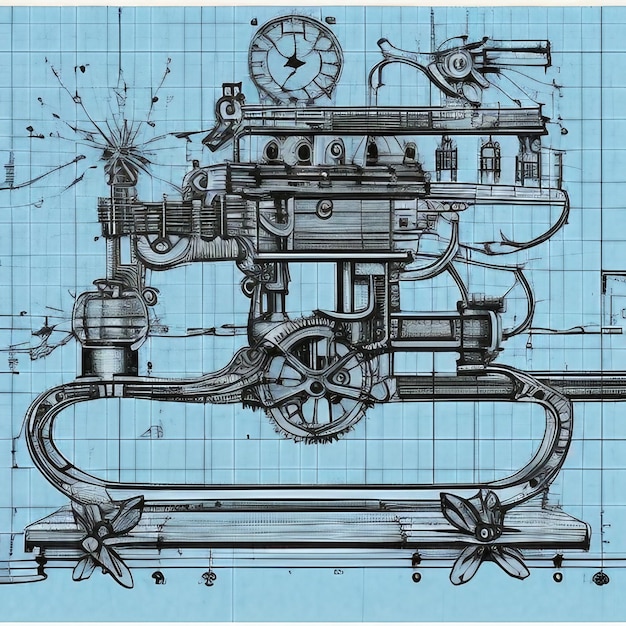The detailed image is a meticulously drawn blueprint of a complex steampunk-inspired machine, set against a blue grid background. The machine, illustrated in gray lines, is an intricate assembly of pipes, gears, valves, dials, tubes, and chimneys. These elements are interconnected, suggesting a fantastical yet non-functional contraption, possibly an artist's imaginative vision of a futuristic device. There is no clutter of colors; the entire sketch maintains a monochromatic scheme with the gray details standing out against the blue background. The machine appears decorative, featuring fans at the bottom and what might be a wooden platform, adding to its stationary and ornamental nature despite the absence of a clear practical purpose. The image exudes a distinctly steampunk aesthetic, blending old-fashioned industrial elements with a touch of whimsy and creative ingenuity.